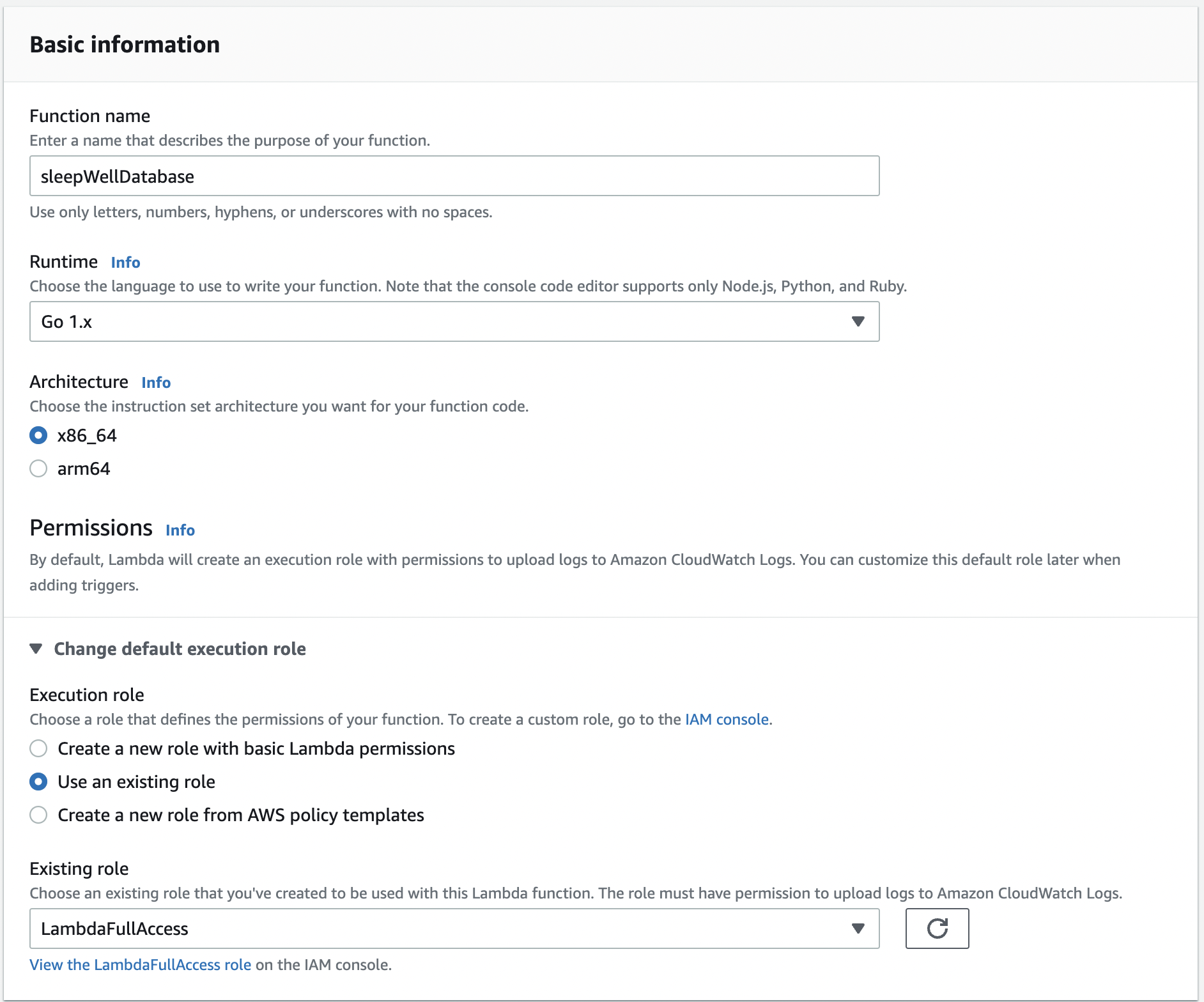The page features a meticulously organized list of functions, set against a pristine white background. All text on the page is rendered in either black or dark gray, depending on whether it is a title, subtitle, or description. Splashes of blue text appear sporadically next to titles and subtitles, labeled "info," which likely offer additional information when clicked. At the very top, the phrase "Basic Information" stands out in a bold, black, sans-serif font, clearly signifying the section's importance. The page is divided into various subsections, each underlined by subtitles reading "Function Name," "Run Time," "Architecture," "Permissions," "Execution Role," and "Existing Role." 

Interaction elements vary across the page: certain functions feature type-in bars for user input, others present drop-down menus for selection, and a few offer lists from which users can choose predefined options. Each design choice caters to making the data entry and selection process intuitive and user-friendly.